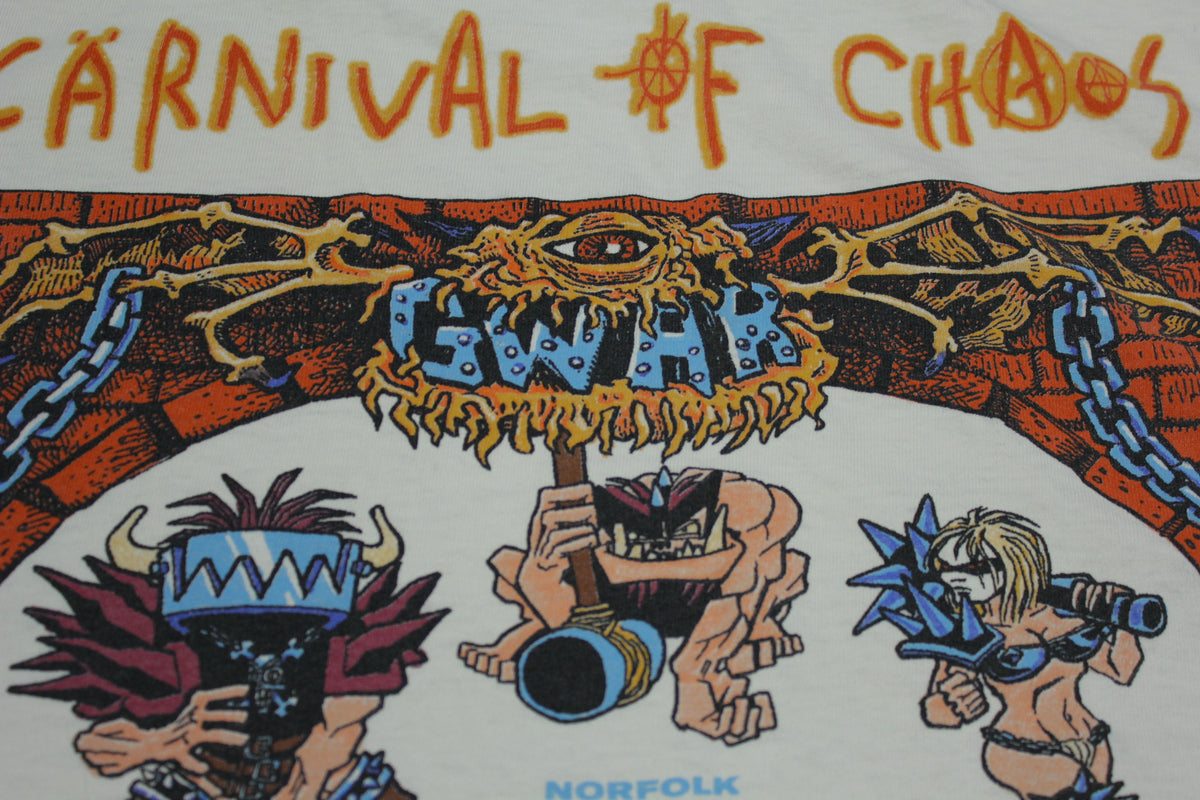This is an album cover or merchandise art for the band GWAR, titled "Carnival of Chaos." The artwork features vibrant, chaotic colors including orange, blue, and burgundy. At the top, "Carnival of Chaos" is scrawled in crayon-like letters with a compass-style "O" in "of." Below is a brick plinth or archway with a central, many-legged monster eye labeled "GWAR." 

Chains radiate from this central figure, and beneath it are three grotesque, cartoon-like characters. In the center, a large monster with giant incisor teeth, massive hands and feet, wields a colossal hammer. To the left, another creature sports a face devoid of features except for jaw-like teeth and bull horns, carrying a skull mask or shield. On the right, a scantily clad woman in a chain mail bikini and glasses holds a mace.

Additionally, the word "Norfolk" is printed at the bottom, suggesting either a concert location or event tied to this artwork. The scene exudes a vivid sense of chaos and fantasy, perfectly fitting for an album cover.